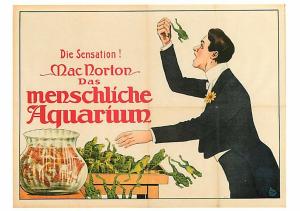This advertisement features a man in a blue suit with a white shirt, a white bowtie, and a yellow flower on his lapel, holding a frog above his face with an expression of surprise. The man's brown hair frames his face as he gazes directly at the frog, which appears to be trying to jump out of his grip. To the left, a fishbowl filled with multiple orange goldfish sits on a table that is swarming with frogs, which are drawn all over and leaping off in various directions. The background consists of a yellow piece of paper bordered in black. Five lines of purple text, in different fonts, appear on the left side of the image, with the red-colored headline reading "Dye Sensation Mack Norton Doss Menschkli Aquarium." The text might be in German or another unfamiliar language. The setting appears chaotic as frogs jump everywhere, capturing a moment of whimsical disorder.